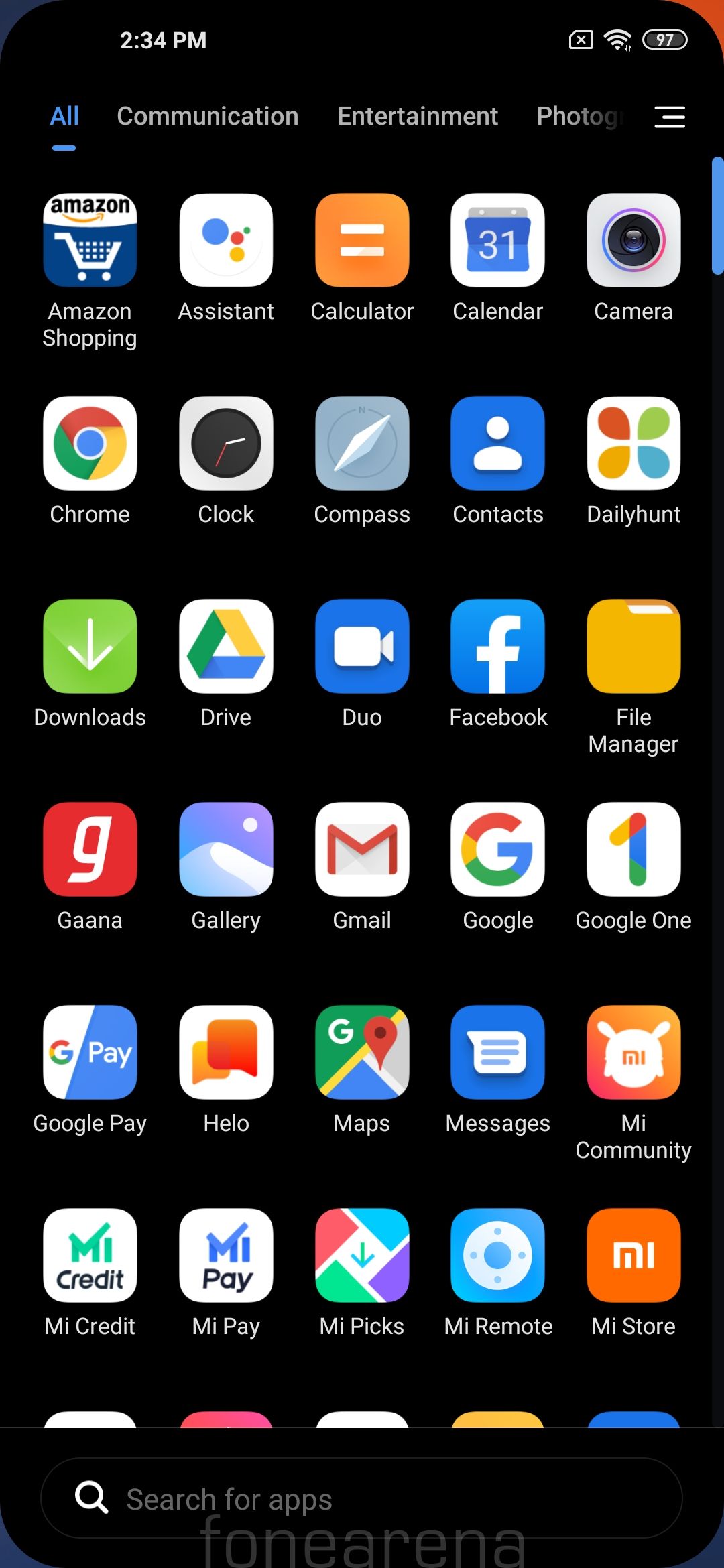The screenshot, taken at 2:34 p.m., features a smartphone interface with a black background and a battery life of 97%. The home screen displays a neatly organized app grid with icons predominantly in shades of blue, categorized under communication, entertainment, and photos. Visible apps include:

- Amazon Shopping
- Assistant
- Calculator
- Calendar
- Camera
- Chrome
- Clock
- Compass
- Contacts
- Daily Hunt
- Downloads
- Drive
- Duo
- Facebook
- File Manager
- Gaana
- Gallery
- Gmail
- Google
- Google One
- Google Pay
- Hello Maps
- Messages
- My Community
- My Credit
- My Pay
- My Picks
- My Remote
- My Store

At the bottom of the screen, a black rectangle houses a search bar with a magnifying glass icon, labeled "Search for apps", and an additional app, PhoneArena, is partially visible. The top of five more app icons is cut off above. The layout exemplifies a well-structured and user-friendly mobile interface.